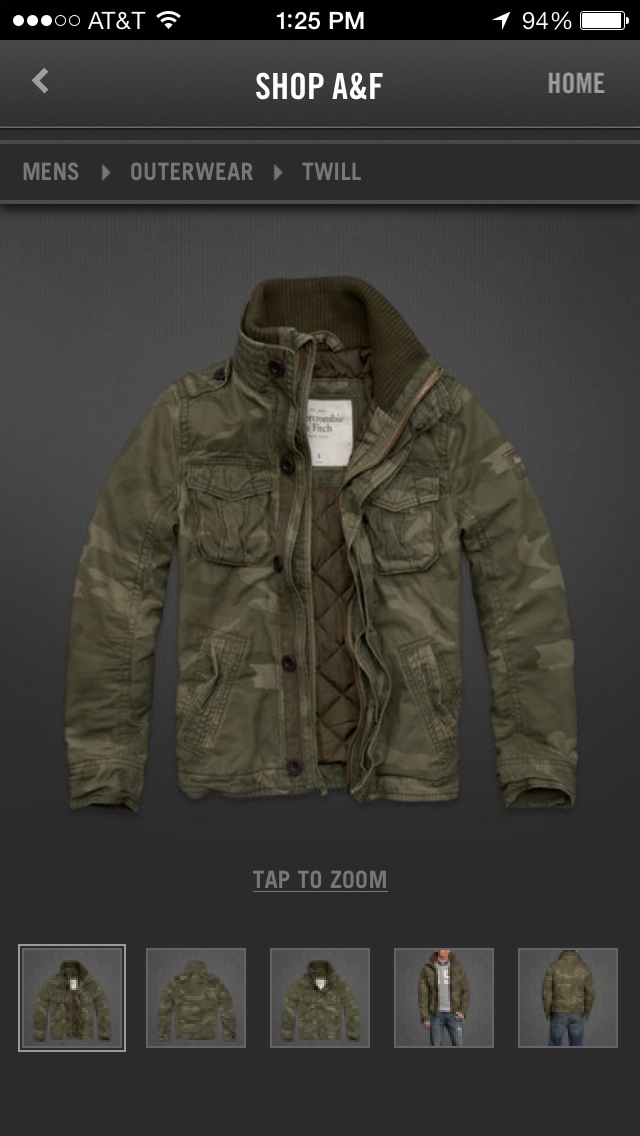The image is a rectangular screenshot of a smartphone displaying a webpage from the Abercrombie & Fitch website. Indicators at the top of the screen reveal it's 1:25 PM, the phone is connected to AT&T with a strong Wi-Fi signal, and the battery is at 94%. The main content of the screenshot focuses on a men's camo long-sleeve outerwear jacket. The header of the webpage reads "Shop A&F" in white, set against a dark gray background. The page indicates the user is browsing the men's department, specifically under outerwear and twill categories. The jacket, prominently displayed in the center of the screen, appears to be heavy and warm with a high collar and zip-up design. Below the main image, the webpage provides a "Tap to Zoom" link and five smaller thumbnails, allowing users to view the jacket from different angles, including the front, back, and on a model.